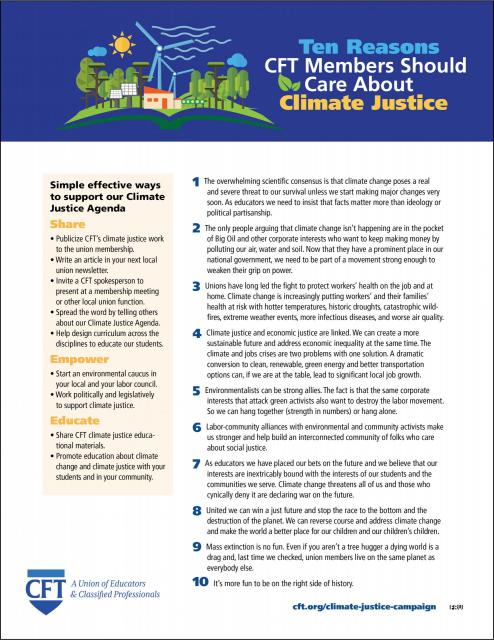This image is a detailed page from a climate justice action document titled "10 Reasons CFT Members Should Care About Climate Justice." It features a visually structured and informative layout. At the top quarter of the page, there's a blue bar, and to the left, an illustration depicted with windmills, solar panels, and other sustainable living icons sitting on an open book that flows into hill-like shapes. The primary headline, "10 Reasons CFT Members Should Care About Climate Justice," is prominently displayed with "10 reasons" in light blue, "climate justice" in yellow, and the remaining text in white. Below this, the main body contains ten bullet points with accompanying short paragraphs elaborating on each reason. 

The left column has a pale yellow background rectangle, providing a subtle highlight for additional information. The top section reads, "Simple Effective Ways to Support Our Climate Justice Agenda," followed by three dark yellow subtitles: "Share," "Empower," and "Educate," each accompanied by their respective bulleted lists containing small black text details on how members can get involved. At the bottom left corner of the page, there's a logo with the initials "CFT," enclosed within a rectangle and a blue triangle, indicating that this is from the CFT, a Union of Educators and Classified Professionals. The document suggests further information can be found at the website, cft.org/climate-justice-campaign. The colors used throughout the page include shades of blue, green, reddish hues, beige, and various yellows, creating a harmonious and engaging design. This setting makes it ideal as a leave-behind sheet for meetings, allowing attendees to reflect on the discussed points.